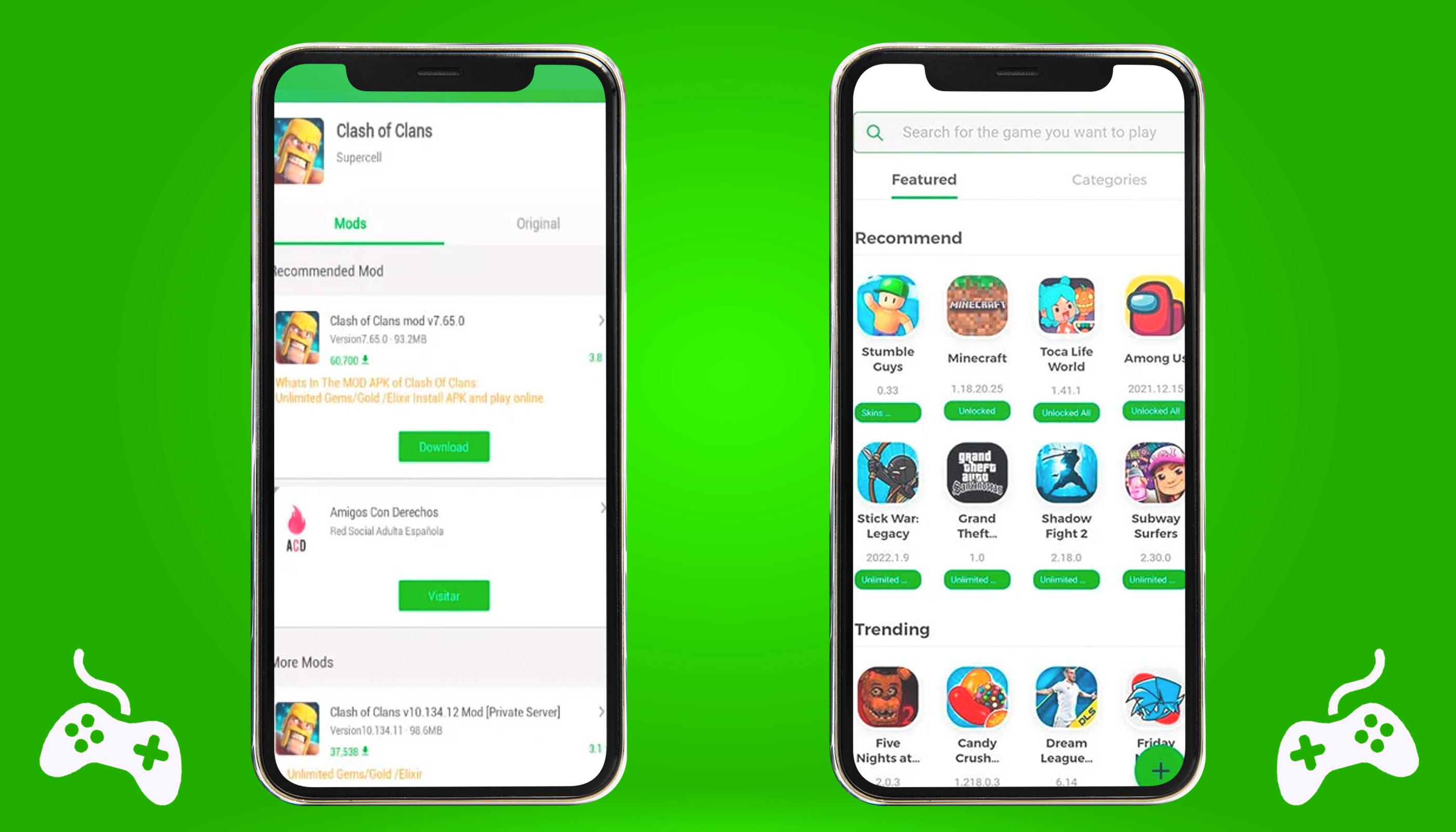The image features a gradient green background that transitions from a lighter shade in the center to a darker hue at the edges. Prominently positioned in the center are two generic looking iPhones displayed side by side. The iPhone on the left shows a screenshot from the game 'Clash of Clans,' specifically highlighting a mod version labeled 'Clash of Clans Mod V7.6.5.0'. The iPhone on the right presents a list of various apps available for download, with sections like 'Recommended,' 'Trending,' and a search bar at the top, reminiscent of an app store interface. In the bottom left and bottom right corners of the image, there are small white gamepad logos, each depicting a traditional controller with a wire extending out of it. The screen captures on the iPhones are quite small, making most of the text illegible. However, the overall composition suggests a focus on mobile gaming apps and downloadable content.